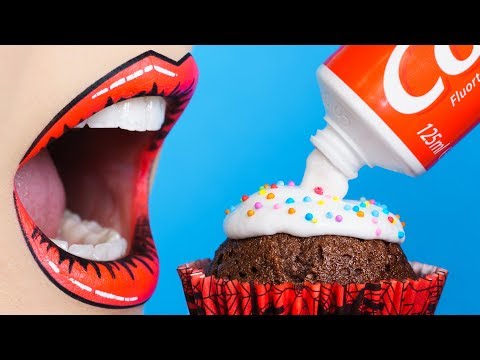The image is a surreal, digitally-created scene depicting a bizarre and playful juxtaposition. On the left side, there's a close-up of a woman's open mouth, with vividly colored, pop-art style lips that look animated or digitally edited, revealing real-looking teeth and a tongue. On the bottom right, there is a chocolate cupcake adorned with colorful sprinkles. The peculiar detail that stands out is the frosting being applied from a toothpaste tube, with the white substance, possibly toothpaste, being squeezed out from a Colgate-like tube hovering in the top right corner. The overall composition has a blend of realistic elements and cartoonish enhancements, creating a striking contrast. The image also features a black frame around the top and bottom, adding to its surreal and artistic feel. The color palette includes red, white, light blue, blue, shiny red, and tan. In the background, faintly visible letters 'C' and 'O' suggest there might be additional context that is hard to read due to the small size.